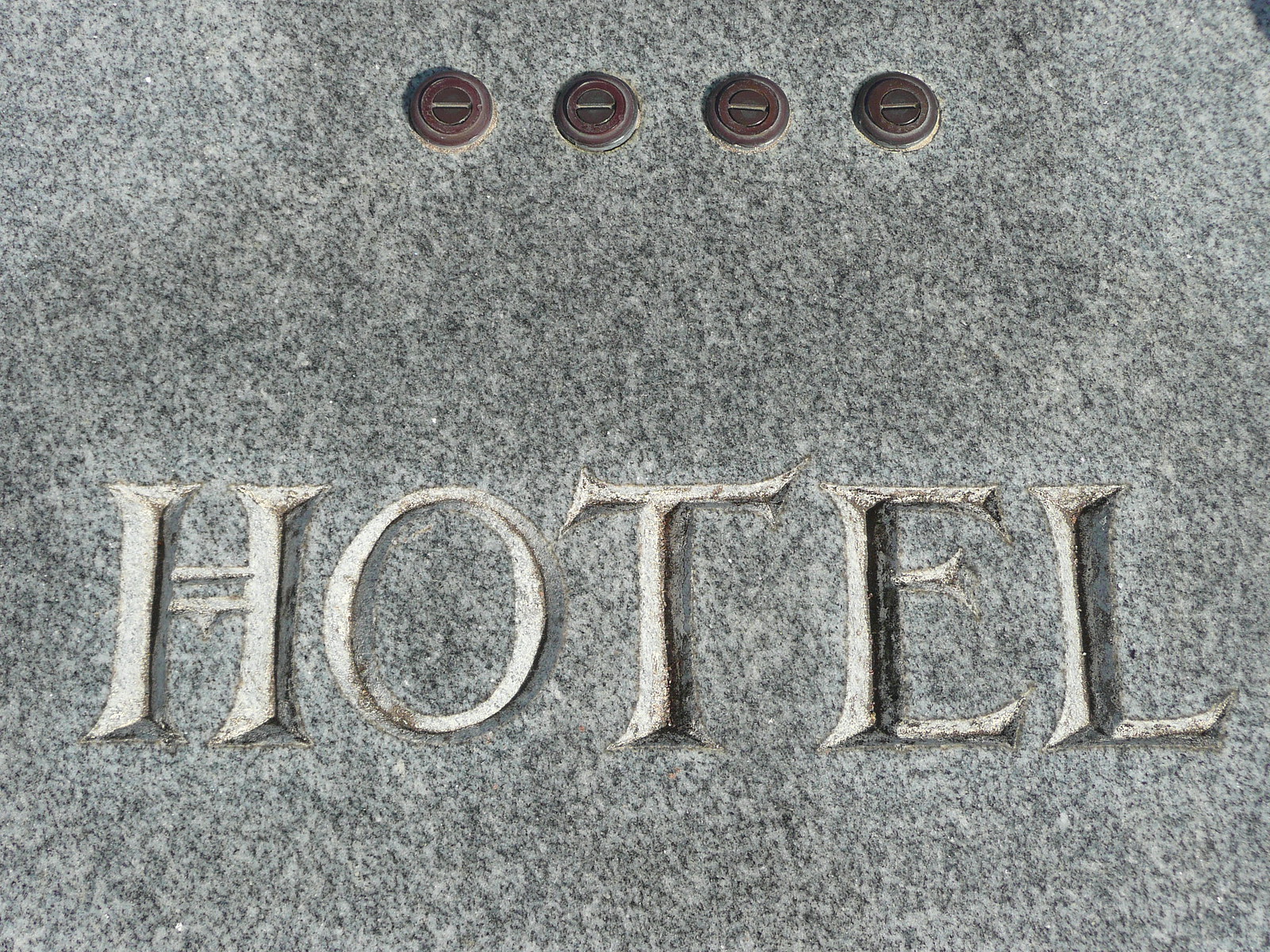The photograph showcases a single large slab of gray granite stone, characterized by its grainy surface adorned with white, black, and gray specks. Dominating the lower half of the image is the raised, three-dimensional word 'HOTEL,' appearing almost ancient and weathered. The white paint on the lettering has worn off at the sharper points and curves, revealing the gray stone beneath and adding to the aged look. At the very top of the stone, there are four circular recesses housing caps that resemble weathered metallic elevator buttons or bolts, their purpose unclear.